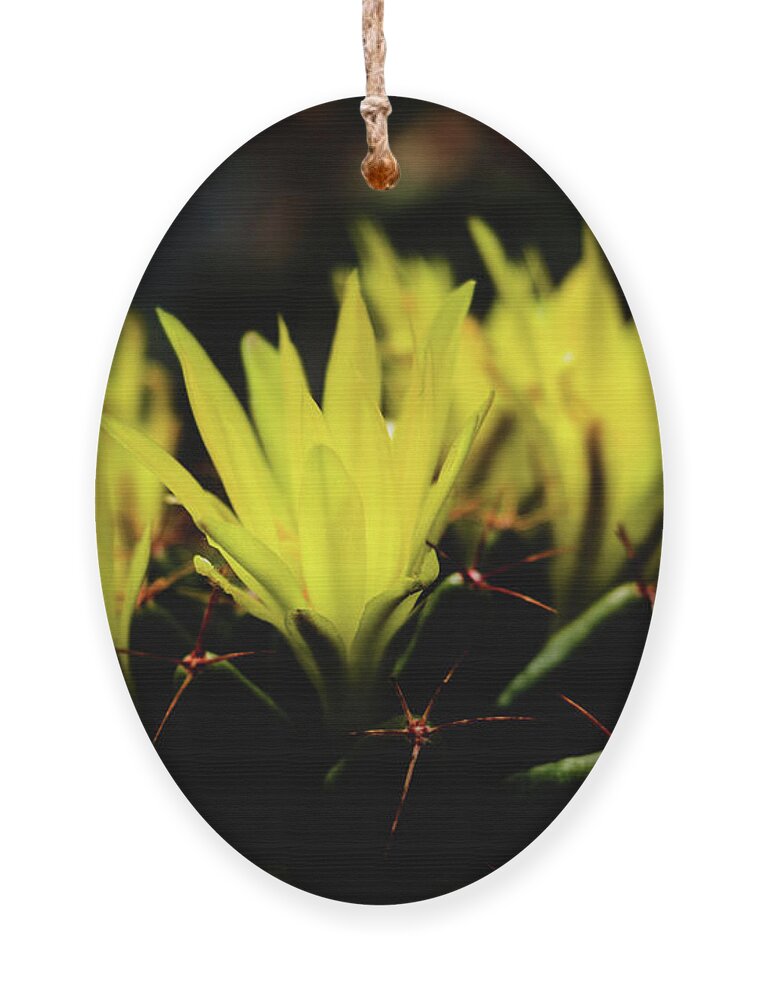The image features a close-up, oval-shaped photograph resembling a hanging ornament, complete with a string looped through a hole at the top. This gives the impression the image could be hung like an ornament. The focal point inside the oval is a partially bloomed yellow flower, surrounded by an array of red, star-shaped thorns grouped in clusters of five. The flower is highlighted by a brighter light in the center, while the background remains dark and blurry. The presence of orange and black thorns adds to the complex texture of the image. The entire setting evokes the feel of a blossoming flower captured amidst a thorny, contrasting backdrop, lending a detailed and intimate view of this botanical scene.